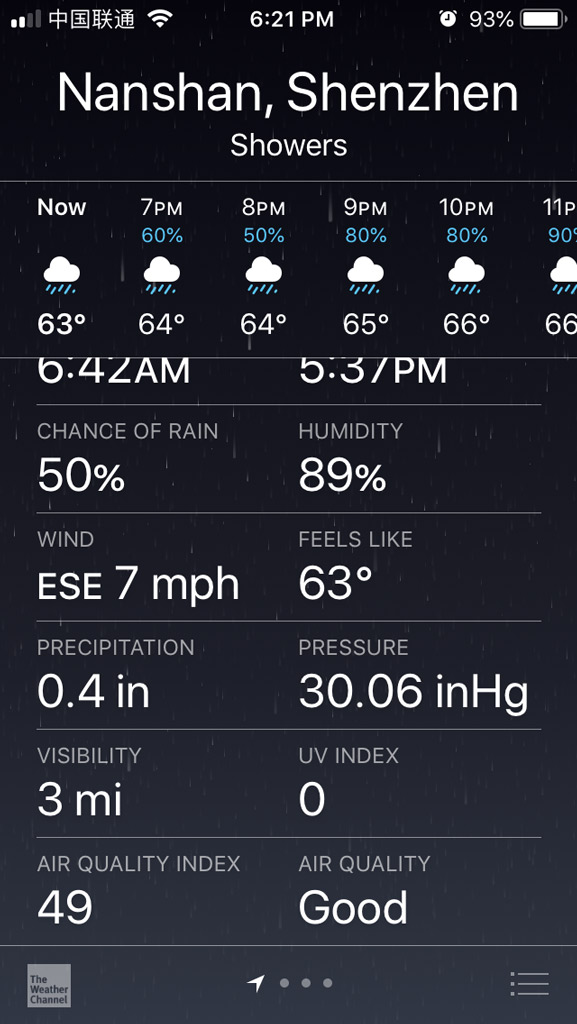The image depicts a weather report for Nanshan, Shenzhen, presented on a dark gray or black background. At the top center, the time "6:21 PM" is displayed in white letters. The top left corner shows a battery life indicator at 93%. 

Below the time, the location "Nanshan, Shenzhen" is written in white lettering, followed by the current weather condition "Showers."

An icon of a white cloud with blue raindrops represents the ongoing rain, accompanied by a text indicating a 63% chance of rain. The hourly weather forecast follows underneath in chronological order:

- 7 PM: 60% chance of rain with a white cloud and blue raindrops icon.
- 8 PM: 50% chance of rain with a similar icon.
- 9 PM: 80% chance of rain with a white cloud and blue raindrops icon.
- 10 PM: 80% chance of rain, again illustrated with a white cloud and blue raindrops.

Further information is provided below these details: 
- "Chance of Rain: 50%" in white letters.
- "Humidity: 89%" in white letters.
- "Wind: East-Southeast at 7 mph" in the same white text.
- "Feels Like: 63°F" is also highlighted in white.

The entire report is formatted against the dark gray or black backdrop for clear visibility of the white and blue text and icons.